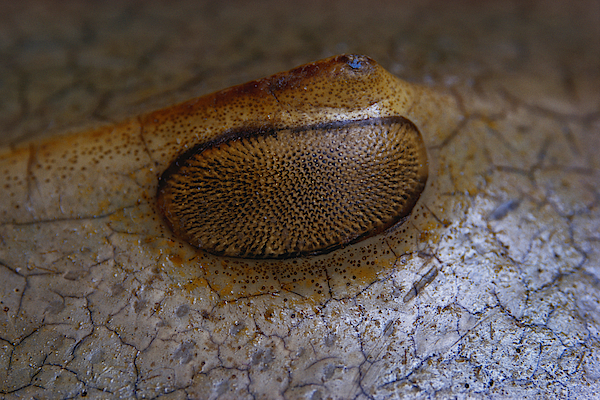The image showcases a close-up, possibly macro photograph, of a non-human surface that evokes an underwater or desiccated environment. Dominating the image is a textured, fissured surface in dark grayish-brown shades, resembling dried, cracked earth. The upper part of the surface is out of focus, contributing to a sense of depth and continuity. Centrally, a pronounced, triangular growth, featuring darker and yellow-brown hues with numerous brown flecks, rises from this surface, forming a notable spine-like ridge. Adjacent to this ridge is an oval-shaped structure with a dark brown, nearly black, outline, and filled with many dark brown to black specks. This structure, ambiguous yet evocative, might be reminiscent of a primitive eye or a peculiar natural formation. The overall color palette is somber, with highlights striking the surface, adding texture and bringing out the intricate details of the image.